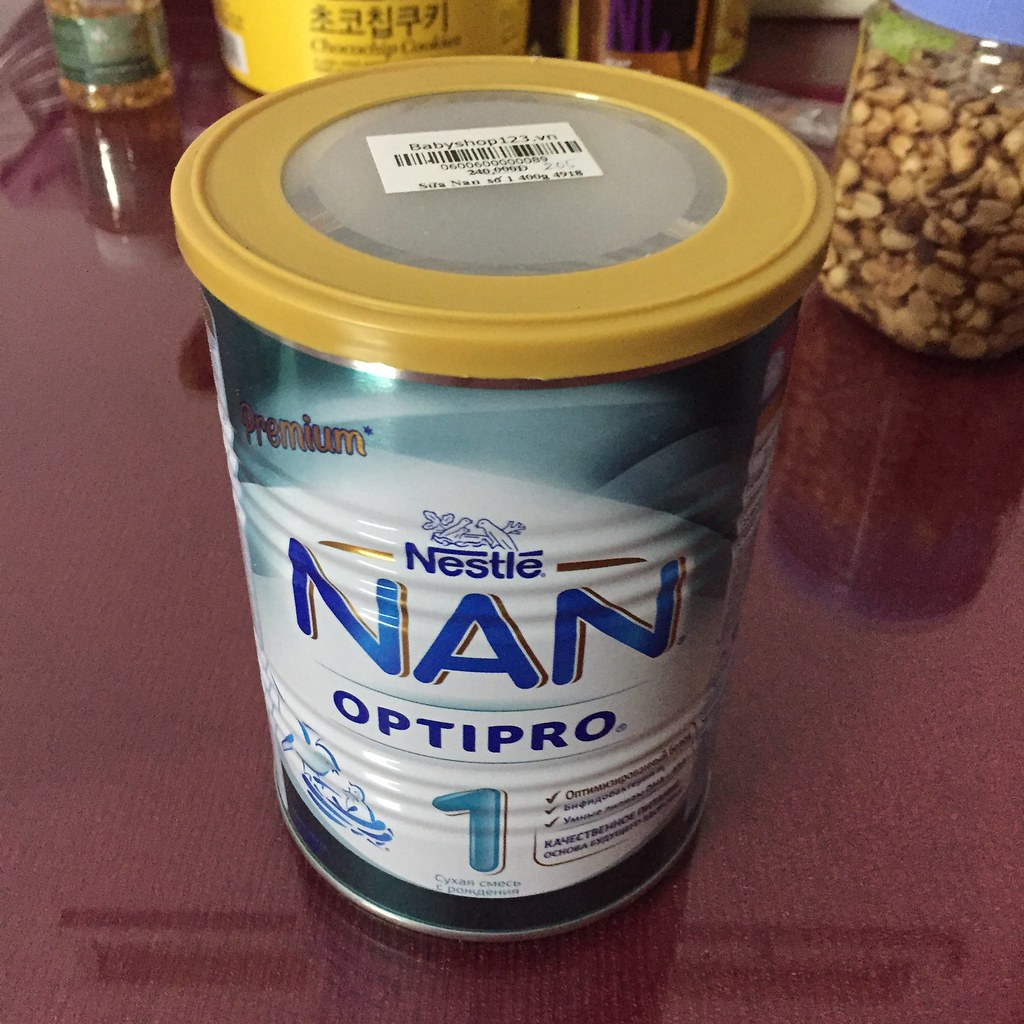In this detailed photograph, the focal point is a close-up view of a Nestle NAN can prominently situated in the center. The can rests on a brown surface, which could be a shelf, table, or countertop. The can itself features a gold lid at the top, followed by a light blue, white, and navy blue body. The text on the can reads "Premium" in gold at the top, followed by "NAN" in bold, capitalized letters. Below "NAN," the word "OptiPro" is visible, and beneath this, the large number "1" is centered on the can's body.

In the upper-left corner of the image, just beyond the Nestle NAN can, part of another can is visible. This secondary can is yellow with brown, possibly Asian, print. Additionally, in the upper right corner of the image, there is a clear jar filled with a variety of mixed nuts, adding depth and context to the scene.